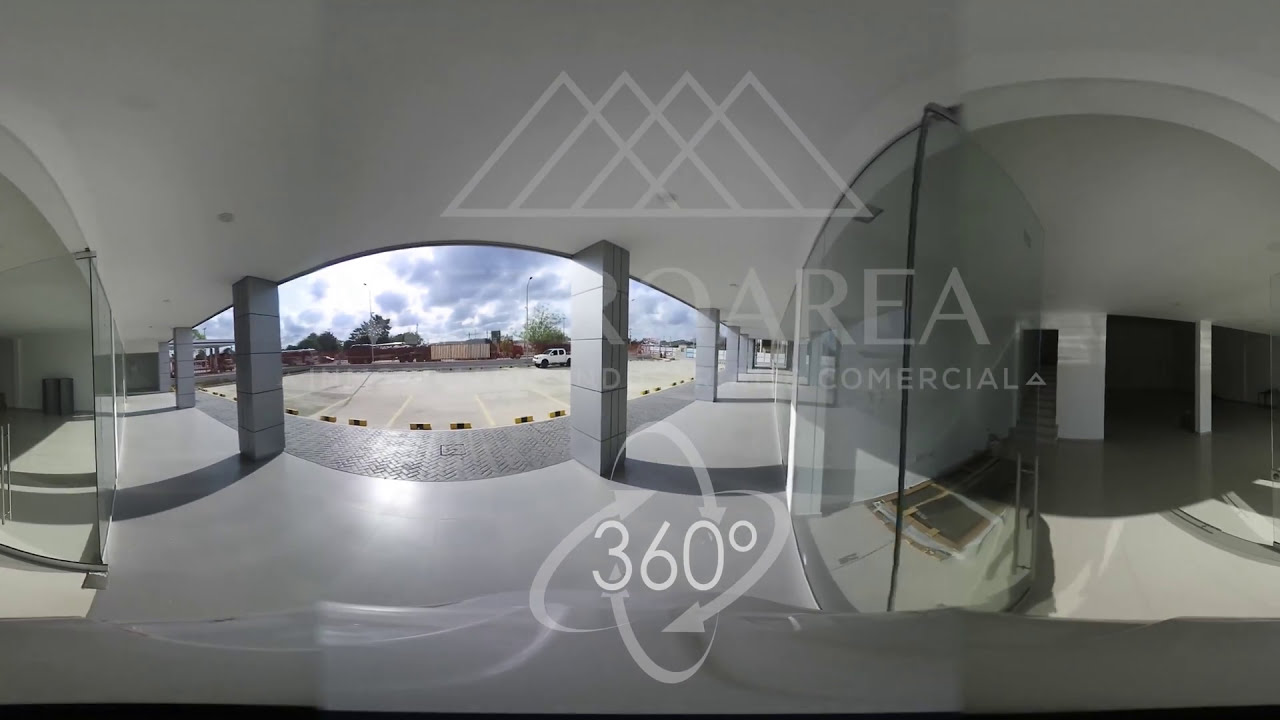The full-color, digitally enhanced photograph features a horizontal rectangle with a thin black border along the bottom. It includes gray text that is difficult to read but appears to say "Rorya Commercial 360" along with arrows illustrating 360 degrees. At the top, a logo resembling a mountain made of triangles is visible. The image captures the inside of a minimalistic building with white floors, white ceilings, and gray support columns. The scene looks out through a large glass wall with doors, revealing a mostly empty parking lot under a visible sky, with a distant white pickup truck as the only vehicle. The setting includes a sidewalk and storefronts, adding to the commercial atmosphere of the area.